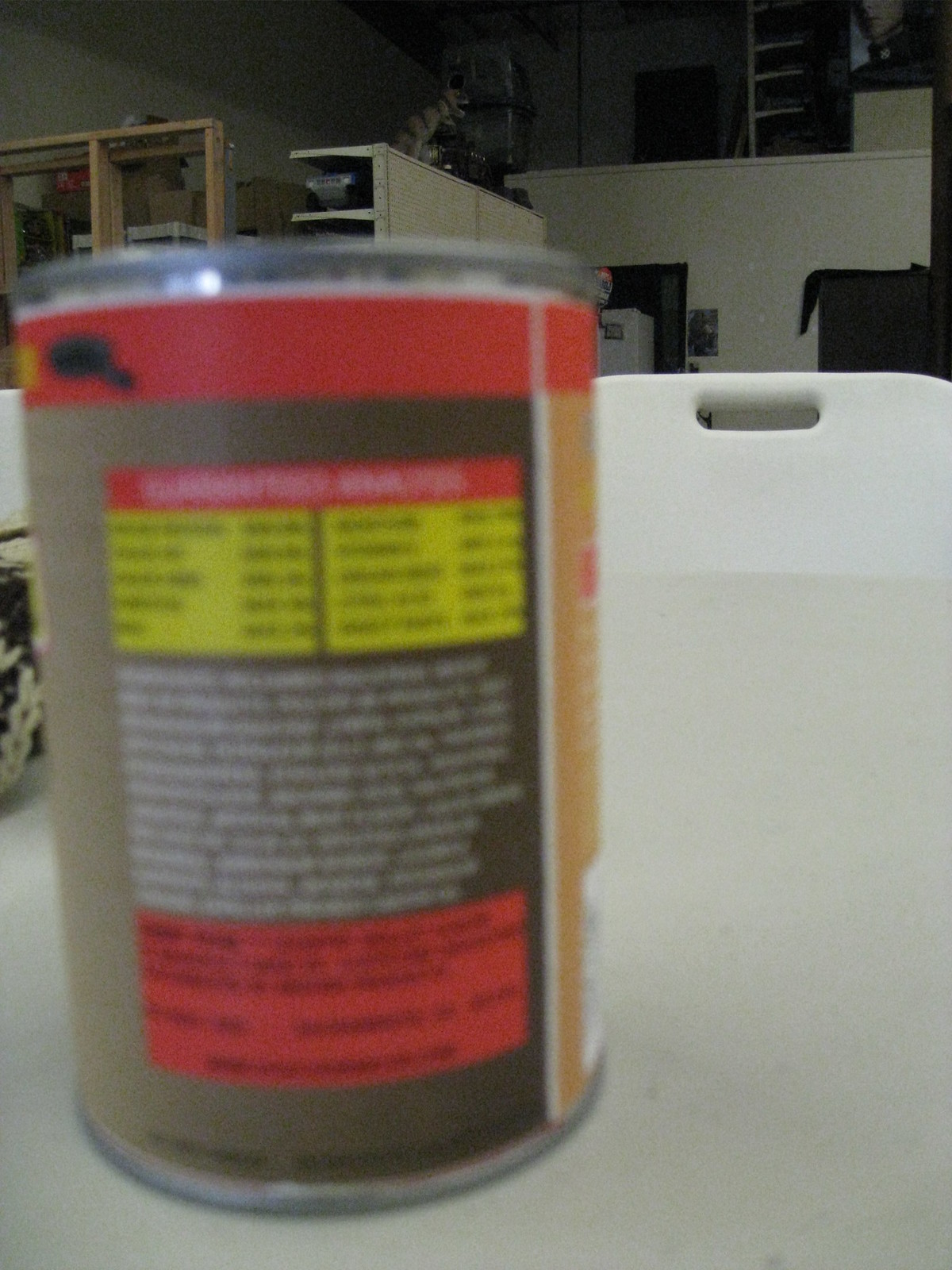In a spacious kitchen, a white table holds a can of food, positioned with its back facing the viewer. The can's design features a dark brown and yellow nutrition label, displaying black text against a yellow background and additional red and white text. The extensive ingredient list stands out in white writing on a black box. A white object, possibly a chair or cutting board, is visible in the background, along with shelving. Another item accompanies the can on the table, adding to the scene's intricacy. The can itself has a light brown label on its front and a plastic top, reflecting its practical and detailed packaging.